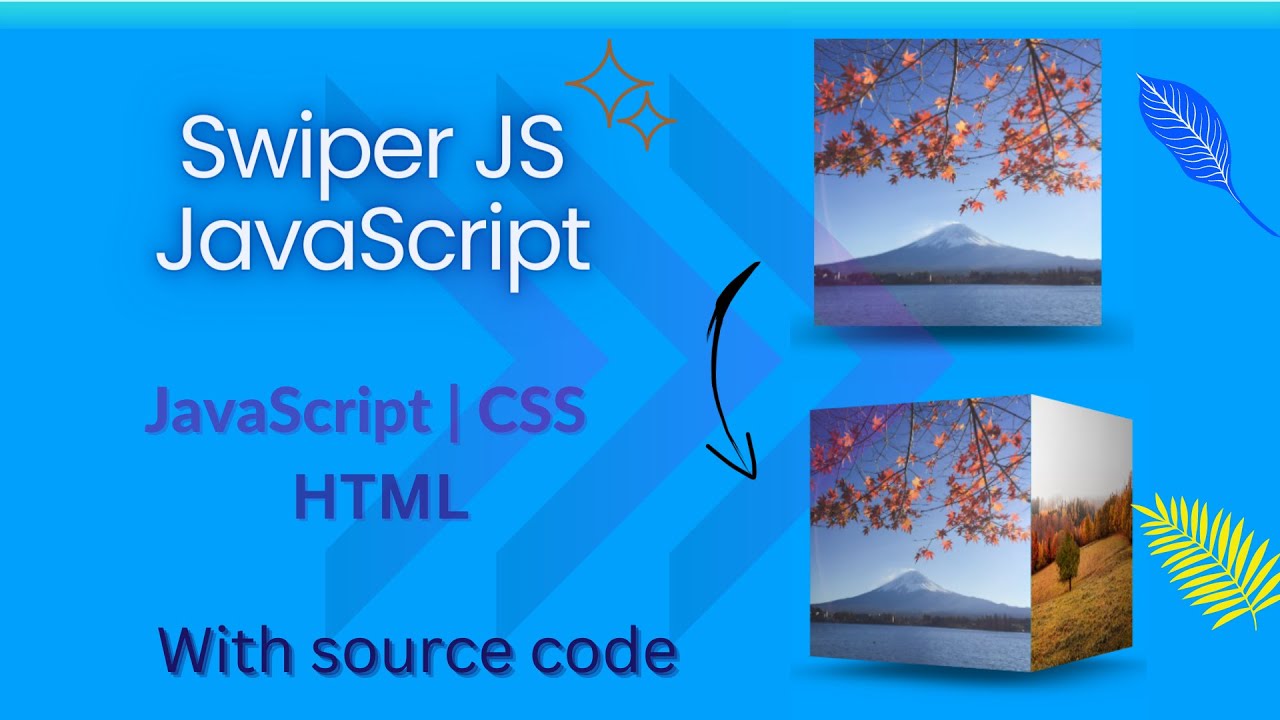In this vibrant image composition, the central theme revolves around SwiperJS JavaScript. The upper section of the image features a white text on the top left corner that reads "SwiperJS JavaScript." Right beneath, there is a smaller text in purple stating "JavaScript CSS HTML." Another text at the bottom, in dark blue, announces "with source code." The solid blue background is adorned with three horizontally aligned arrows pointing to the right. 

To the top right, a stylized flower leaf is depicted in blue and white, while a similar floral element in striking yellow appears on the bottom right. Central to the design is a square image capturing a branch of a tree dotted with yellow, dried-out, and brown leaves. This picturesque scene is complemented by a majestic, volcano-like mountain in the background with a snow-capped summit fading into a darker base, and a tranquil lake resting below it.

The bottom portion of the image showcases a sliding transition effect; the original image is shifting to the left, thereby introducing another image on the right. This newly revealed image depicts a slope adorned with trees, predominantly yellow highlighted by the light, transitioning into darker hues in some areas. A black arrow from the top image subtly points down to this emerging image below, connecting the visual elements cohesively.